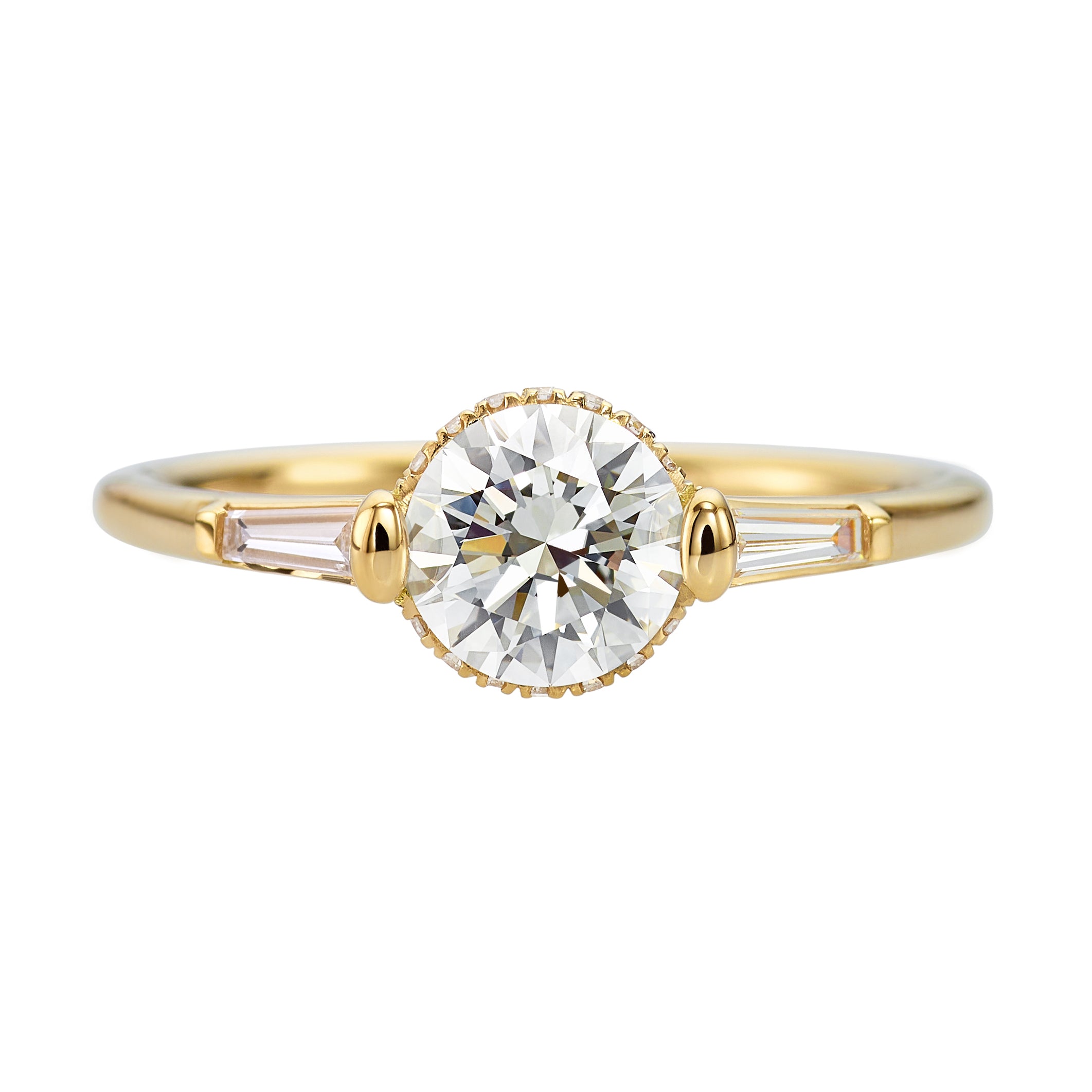The image showcases a close-up, detailed color illustration of an elegant diamond ring set against a pristine white background. The ring, rendered in a landscape orientation, features a radiant circular diamond at its center, which is accented by a sculpted gold rim. This central stone displays a mesmerizing array of prisms in gray, gold, and white, reflecting light and creating a striking visual effect. On either side of the diamond, vertical elliptical gold shapes flank the stone, intersected by angled rectangular diamond shapes that seamlessly connect the central setting to the band. The band itself, in a bright gold finish, exudes a luxurious shine, enhanced by the play of light on its surface. This photographic representationalism captures the ring with all its intricate details and highlights, creating a compelling and elegant product illustration.